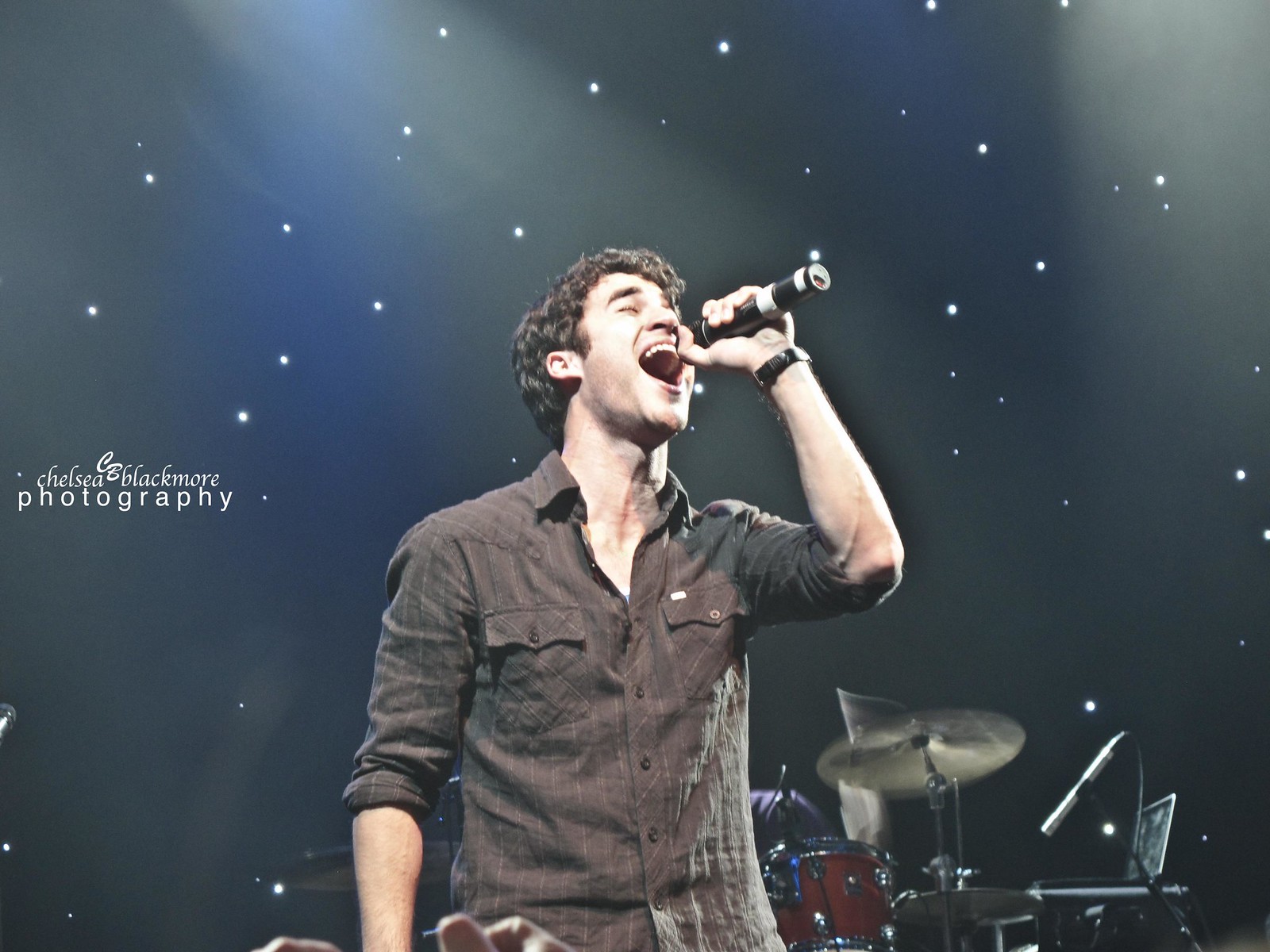In this image, set against a space-themed backdrop with black curtains dotted with star-like lights, a man in his 30s stands center stage passionately singing into a microphone held in his left hand. He has light to dark brown hair and wears a brown cowboy-style button-down shirt with rolled-up sleeves and two breast pockets. His mouth is wide open, revealing his upper teeth as he looks upwards. Behind him, a drum kit is visible, featuring a maroon tom drum, hi-hat cymbals, and various other cymbals. In the bottom left corner of the image, the text "Chelsea Blackmore Photography" is clearly visible in white. The scene appears to be indoors, likely capturing a moment from a live concert.